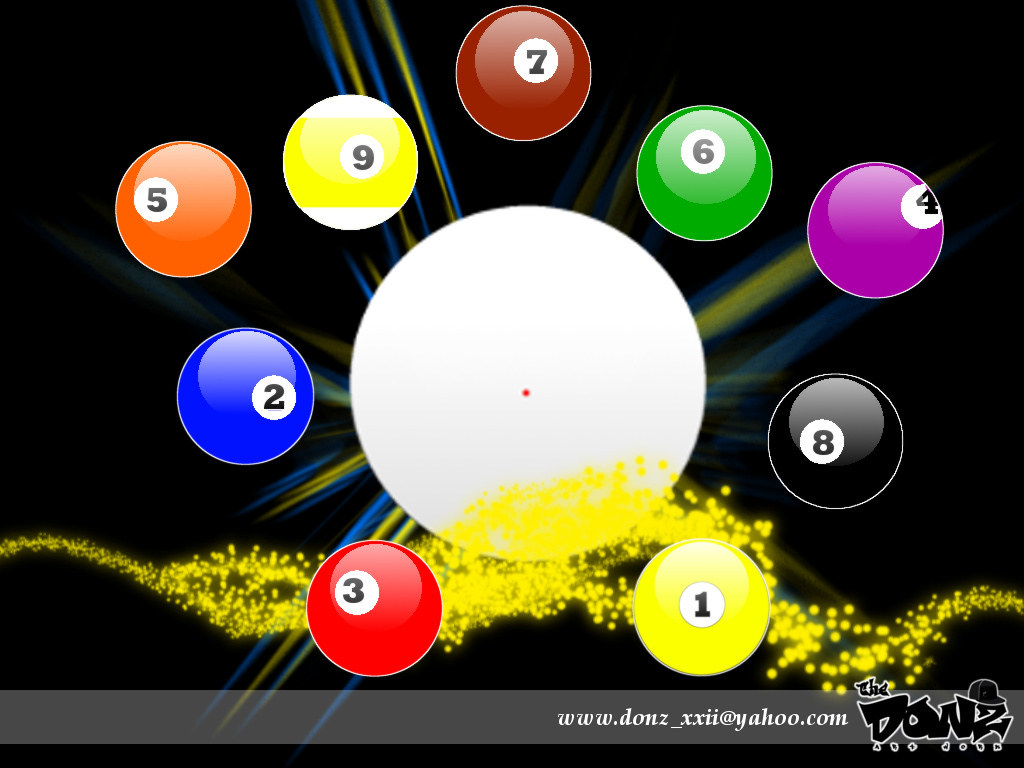This vibrant and detailed illustration advertises a pool or snooker-themed business. Set against a predominantly black background accented with shimmering blue and yellow rays, the image centers around a massive white ball with a tiny red dot in its center, symbolizing the cue ball. Surrounding this white cue ball are the solid-colored pool balls arranged with distinctive colors: the 1 ball in yellow, 2 ball in blue, 3 ball in red, 4 ball in purple, 5 ball in orange, 6 ball in green, 7 ball in maroon, and the 8 ball in black. Notably, the 9 ball stands out with its iconic yellow stripe in the middle and white at the top and bottom. In the lower section of the illustration, a silver or grey strip displays an email address, "www.donz__xxii.yahoo.com," and a business logo labeled "The Donz." The image has an overall neon-like brightness, featuring glittery gold details from right to left, enhancing its eye-catching appeal.